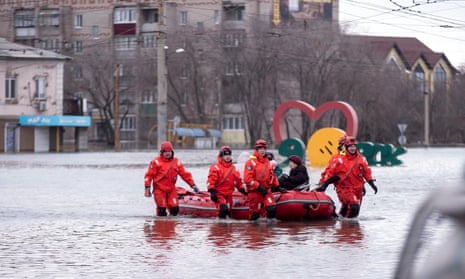The photograph captures a dramatic daylight scene in a flooded city, where a team of rescue workers, clad in full red uniforms and knee-high black boots, are valiantly pulling a red rubber dinghy towards the shore. The dinghy appears to carry elderly women, rescued from the high waters surrounding them. The background displays a large, partially submerged mural featuring a red heart, a green circle, and a yellow smiley face, along with indistinct letters, adding a poignant touch to the scene. Behind the mural, high-rise buildings and trees stand with their lower floors inundated, emphasizing the scale of the flood. The rescue workers are facing the viewer, moving with determination towards the bottom right of the image, as they guide the raft and its occupants to safety.